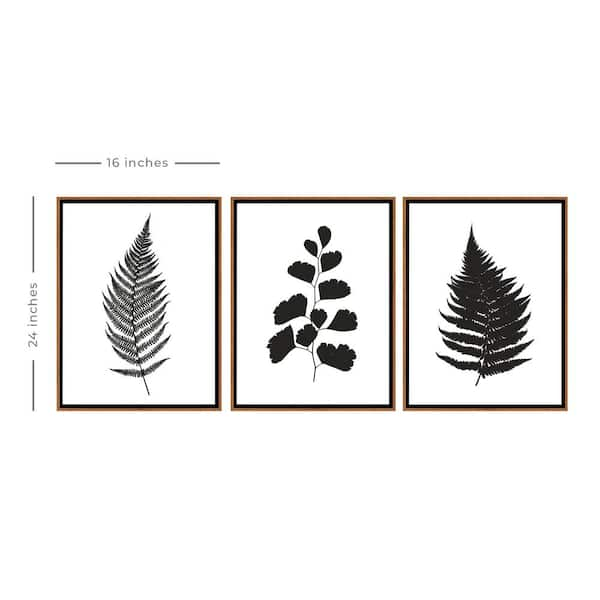The display features three framed, black-and-white artistic depictions of plant leaves, organized in a horizontal row. Each frame is a thin, rust-brown rectangle, uniformly sized at 16 inches wide and 24 inches high. The leaves, presented as dark silhouettes, create a striking contrast against the light background. The image on the left showcases a delicate fern with individual tiny leaves that curve slightly to the right. The middle image presents a larger plant with fanned leaves that are pointy at the bottom and rounded at the top, all connected by a central stem. The right image depicts a thicker fern with broader, darker leaves that curve gently to the left, characterized by more pronounced rounded edges rather than individual leaves. Each frame captures the essence of the leaves' natural structure, giving them an almost tree-like appearance due to their tapered shapes and heavier bases.